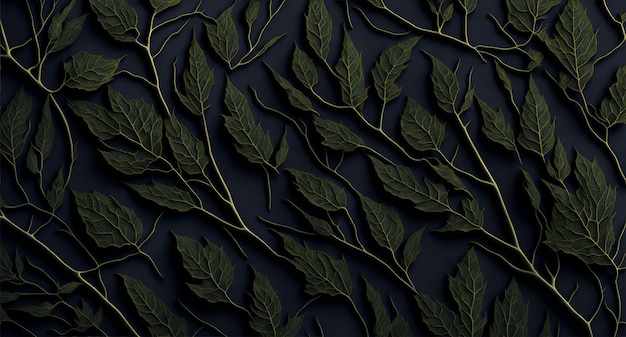This image features a dark, possibly black or gray background adorned with an intricate pattern of green leaves with white stems. The leaves, which vary slightly in shape and size, are distributed throughout the composition, creating a detailed and engaging visual texture. Notable among them are a few larger leaves—one prominently positioned in the bottom right corner and another in the center. The leaves appear darker, perhaps with hints of brown, and each casts a subtle shadow, adding depth and dimension to the scene. This clean, well-organized arrangement suggests a digitally generated graphic, possibly intended as a desktop background or a decorative pattern, and seems to be part of an artistic presentation created in a well-lit setting.